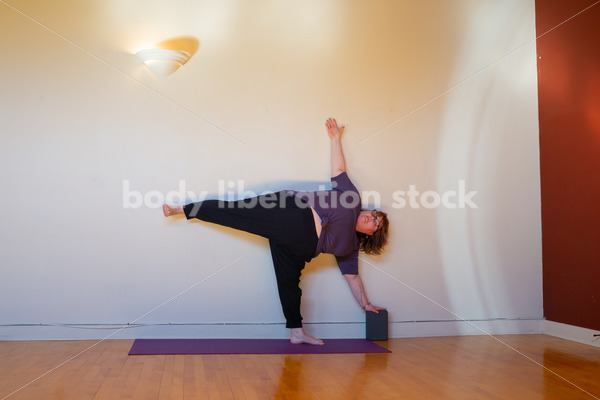This is a detailed photograph of a larger woman performing a yoga pose on a wooden floor. The setting appears to be a bright, possibly a beige or creamish white room, with a distinct light fixture casting shadows that create yellowish and orangeish hues on the walls. The woman is using a purple rectangular yoga mat that matches her purple yoga shirt. She is wearing black yoga pants and eyeglasses. 

In the pose, she forms a 90-degree angle with her legs: her left leg is firmly planted on the mat while her right leg is extended horizontally, forming an L-shape with her body. Her left hand is balanced on a gray rectangular yoga block, supporting her weight, while her right arm is extended straight up towards the ceiling, creating a cross-like silhouette. Her head is turned sideways, and her long brown hair cascades down along her body. She also sports a gold bracelet and appears to have a tattoo along the inside of her forearm. Across the image, there is a watermark that reads "Body Liberation Stock" in white letters.